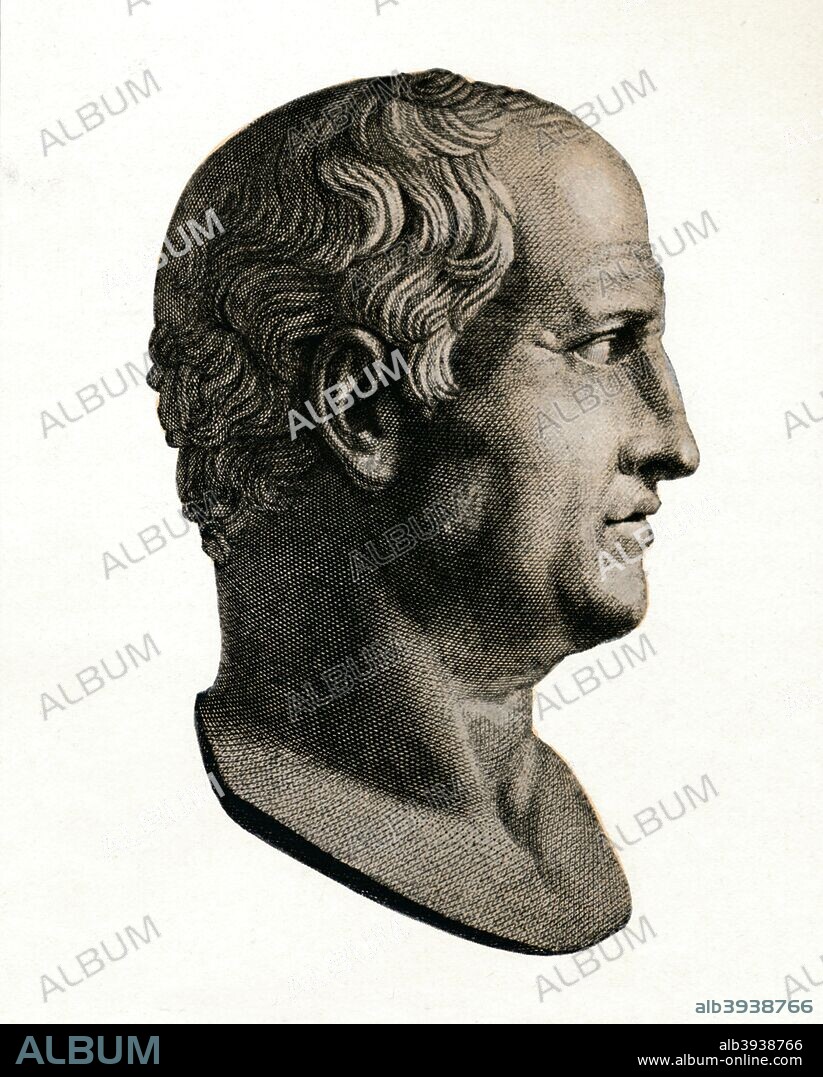This is a meticulously detailed photo illustration featuring the bust of Cicero, renowned Roman statesman and orator. The sculpture is oriented towards the right side of the frame, presenting a profile view that captures the intricate details of his facial features. Cicero's short, white hair is carefully sculpted, and his expression appears contemplative but neutral, reflecting his stoic demeanor. The background of the image is stark white, which emphasizes the classical purity and highlights the texture of the bust. Towards the bottom of the image, a black stripe spans the width with the word "ALBUM" inscribed in prominent blue letters. Additionally, the watermark "album" features prominently on the photo. Along the sides, the text "ALB 393-8766 www.album-online.com" is displayed in neat white lettering, indicating the source from which the image can be accessed. This professional arrangement ensures that every element, from the historical significance of Cicero to the modern informational text, is presented in a balanced and visually appealing manner.